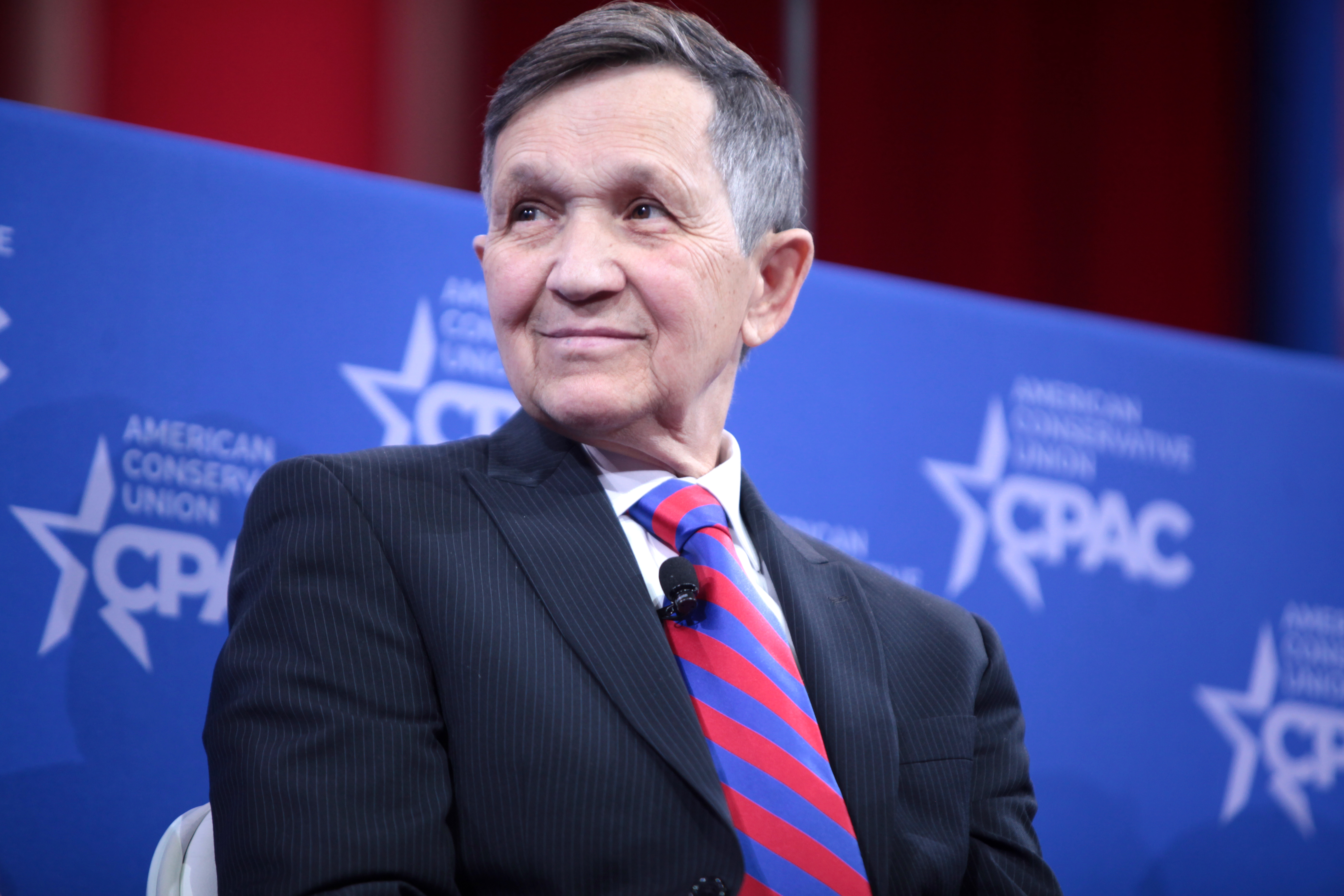The photograph captures an older gentleman seated on a white chair, exuding a dignified presence that suggests he might be a politician. He sports a dark pinstripe suit paired with a bold red and white diagonal striped tie, to which a wireless microphone is clipped. His dark hair, graying at the sides and slightly on top, is neatly parted to the left. The man's face is lined with wrinkles, particularly around the eyes, and he offers a slight, knowing smile while gazing to his right, which is the left side of the image. Dominating the background is a royal blue banner emblazoned with the white text, "American Conservative Union" and the CPAC logo, set against a red wall, hinting at the event's formal setting. The repeated star logo in front of the "C" in CPAC punctuates the significance of the gathering.